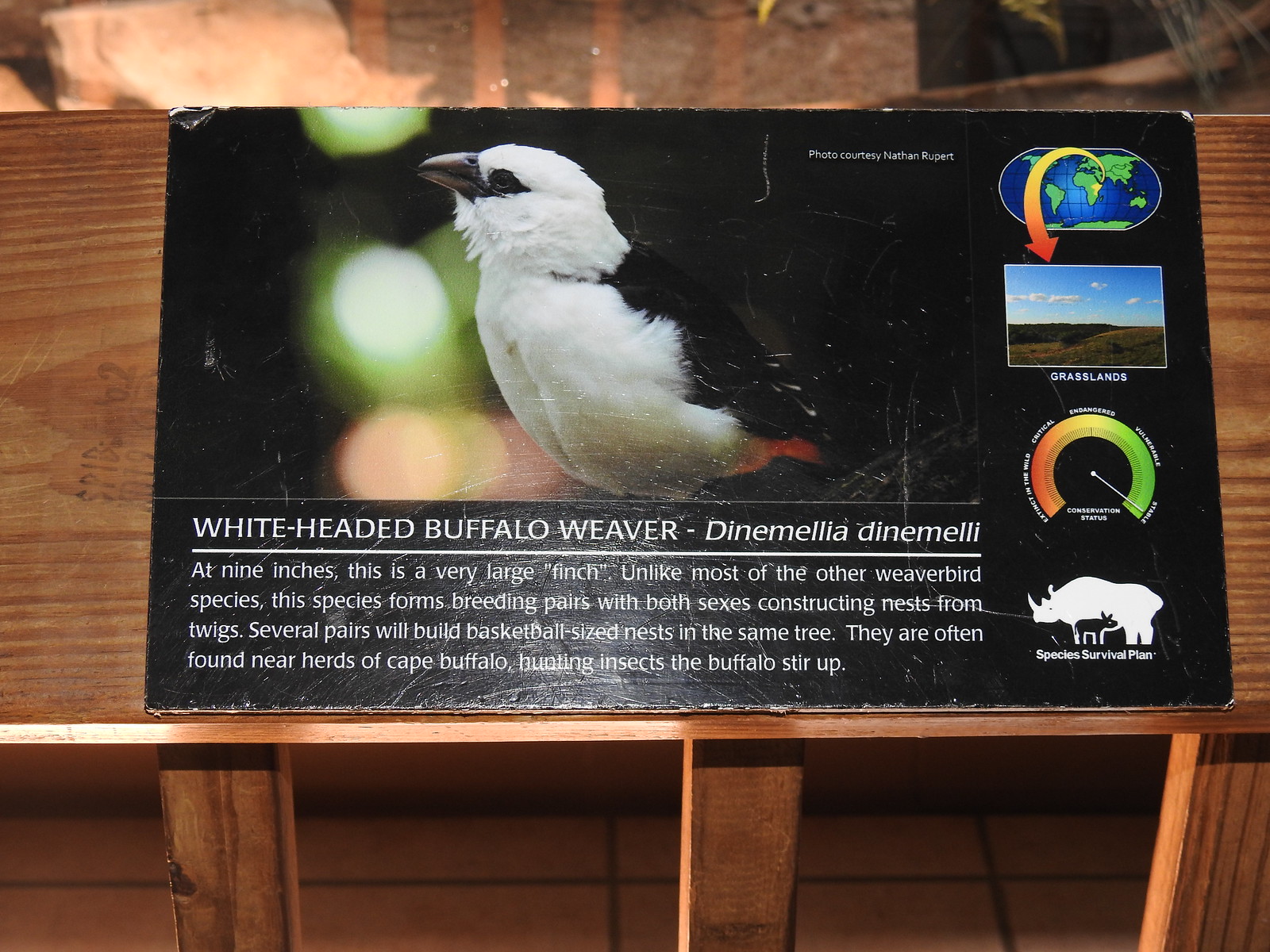The image features an informational sign affixed to a wooden background, likely within a zoo or national park. The sign's worn edges and scuffed surface suggest frequent handling and exposure. The sign itself has a black background, with a prominently displayed photograph of a white-headed buffalo weaver (Dynamelea dynamele) at its center. The bird, looking to the left, is primarily white with black feathers on its back, a black eye, and a black beak.

Beneath the bird’s image, white text provides detailed information about the species: "The white-headed buffalo weaver, Dynamelea dynamele. At nine inches, this is a very large finch. Unlike most of the other weaver bird species, this species forms breeding pairs with both sexes constructing nests from twigs. Several pairs will build basketball-sized nests in the same tree. They are often found near herds of Cape buffalo, hunting insects that the buffalo stir up."

To the right of the bird’s photo, the sign includes several smaller images and icons arranged vertically: an illustration of the continents indicating the bird’s range in Africa, a photograph labeled "grasslands," a climate dial, and finally, a silhouette of rhinoceroses with the text “Species Survival Plan” in white. The sign is positioned at the center of a wooden structure resembling a banister or a fence, with colors including black, white, green, orange, and blue, presenting a casual and informative style typical of educational displays.